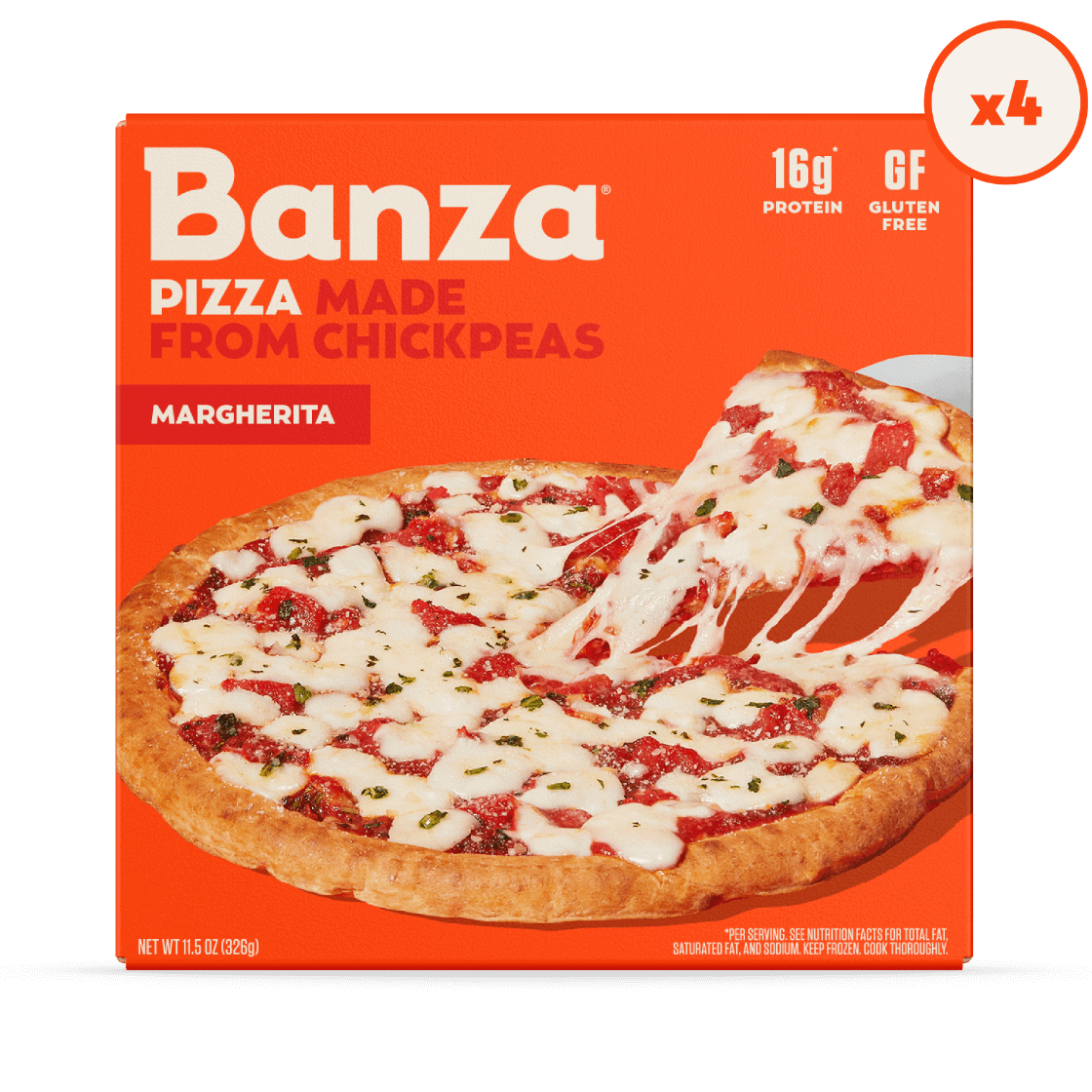The image displays a vibrant orange pizza box for Banza, a brand known for its unique pizza made from chickpeas. Prominently featured in white font is the brand name "Banza" followed by "Pizza made from chickpeas" and the flavor "Margherita." The box showcases a tantalizing image of a whole Margherita pizza with a chickpea crust, adorned with red sauce, mozzarella cheese, and scattered basil leaves, with one slice being lifted to highlight the gooey cheese pull. Nutritional highlights are indicated on the top right, stating "16 grams protein" and "Gluten-free," with a notable white circle with a red outline marked "X4," possibly suggesting a bundle offer. Additional details include the net weight at the bottom left, listed as 11.5 ounces (326 grams). The design hints at providing health-conscious options, reinforced by the "information per serving" notice at the bottom.